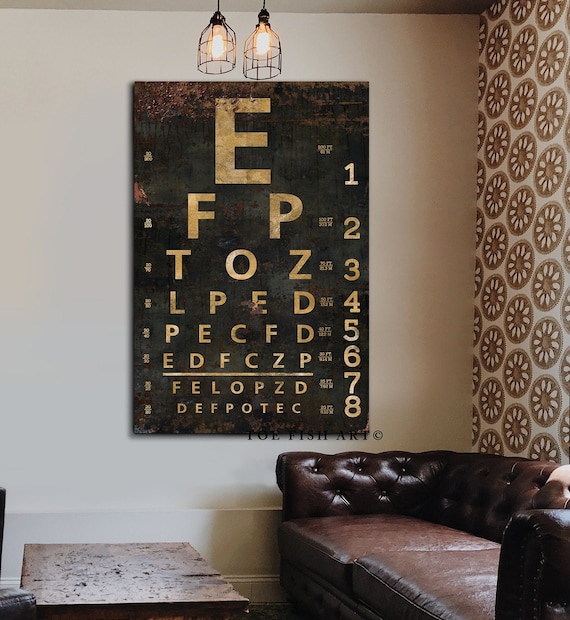The photograph depicts what appears to be a waiting room, possibly of an eye doctor’s office. The room has a beige wall and a section of wallpaper with a brown and white floral pattern on the right side. At the corner where the two walls meet, an old, large eye chart hangs on a dark brown wooden plank. The chart has eight rows of letters, starting with a large "E" at the top, followed by smaller letters: F-P, T-O-Z, L-P-E-D, P-E-C-F-D, E-D-F-C-Z-P, F-E-L-O-P-Z-D, and concluding with the smallest letters, D-E-F-P-O-T-E-C. 

Below the eye chart is a distressed brown leather sofa with plush buttons creating indentations across its surface, adding a touch of vintage charm. In front of the couch stands a worn brown coffee table, possibly made of wood or with a stone tabletop. 

Two light fixtures with wire enclosures hang from the ceiling, illuminating the chart with their warm light. The overall setting combines elements of warm beige, brown, and yellow tones, accentuating the vintage and cozy ambiance of the room.